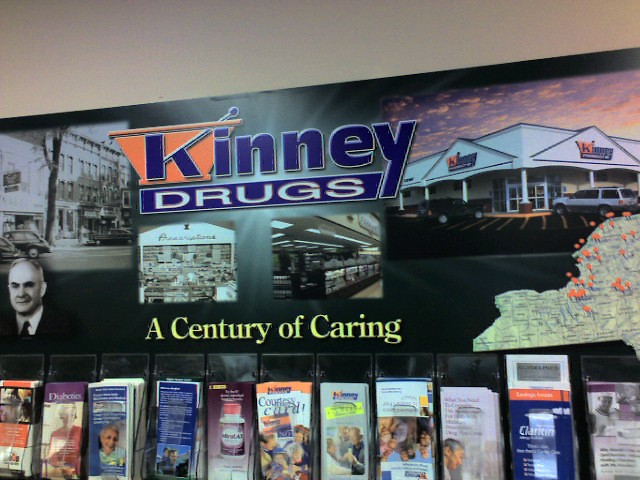The image is of a long rectangular poster hanging on a white wall. The poster prominently features the text "Kenny Drugs" along with the Kenny Drugs logo, where the "K" is stylized within a compound bowl design with a silver stick protruding from its side. The background of the poster is composed of various photos, each with its own thematic element. 

To the left of the poster is a large black-and-white photograph showcasing a significant moment. 

In the center, directly below the Kenny Drugs logo, are two small square photos. The photo on the left is a black-and-white image, presumably of the original pharmacy. The photo on the right features a partial store shot, giving a glimpse into the store's interior.

A large picture on the top left corner of the poster displays the exterior of a Kenny Drugs building, giving context to the brand's physical presence.

In the bottom right of the poster, there is a detailed map dotted with pin markers, indicating multiple Kenny Drugs locations.

Below the poster, a row of different brochures is neatly arranged in plastic holders, spanning from the left to the right, offering additional information and resources.